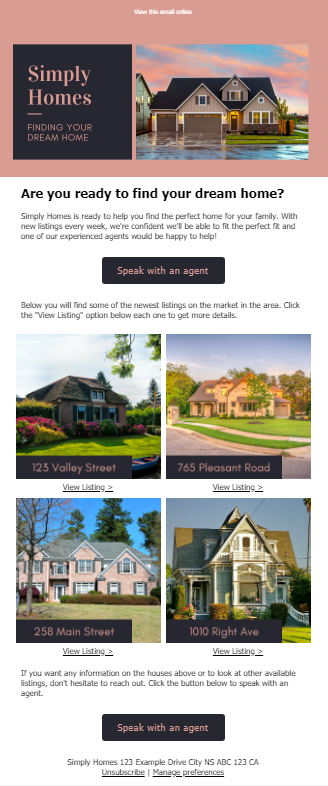### Descriptive Caption:

This image captures a detailed mock-up of an email being viewed on a smartphone. The email, seemingly from a real estate company named "Simply Homes," begins with a soothing mauve header and a dark blue sidebar on the left. Dominantly positioned in the email is the company logo and slogan: "Simply Homes – Finding your dream home."

Beneath the header, an inviting photograph of a charming family home is presented. The home features a two-car garage, situated on a corner lot with wet streets reflecting mauve and pinkish clouds in the background, evoking a serene post-rain atmosphere.

The main content of the email enthusiastically asks, "Are you ready to find your dream home?" It promises assistance from Simply Homes in finding the perfect family abode, showcasing their confidence in weekly new listings. A call-to-action button labeled "Speak with an agent" is prominently placed below this introductory message.

Further down, the email highlights four attractive home listings, each accompanied by a photograph. The homes vary in style, from Victorian with steep roofs and a charming balcony to modern, expansive properties with large lawns. The listings include:
1. 123 Valley Street
2. 765 Pleasant Road
3. 258 Main Street
4. 1010 Wright Street

Each image is followed by a snippet of listing information, prompting viewers to click for more details. Concluding the email, another call-to-action button invites recipients to speak with an agent and underscores Simply Homes' contact details: Simply Homes, 123 Example Drive, City, NSABC, 123 California. Options to unsubscribe or manage email preferences are provided at the very bottom.

This mock-up serves as a polished example of how Simply Homes effectively communicates its offerings and engages potential home buyers through visually appealing and informative email design.